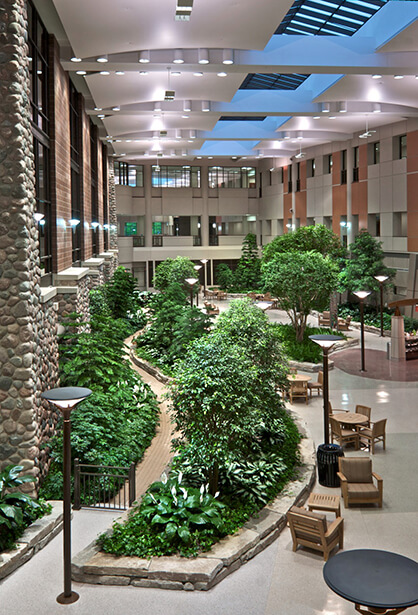This color photograph captures the interior atrium of an office building, showcasing an intriguing blend of indoor and outdoor elements. The high ceiling is adorned with recessed lighting, and large glass windows frame the upper part of the atrium, allowing natural light to filter through. Scattered throughout the space are numerous green trees and shrubs, creating a lush, verdant atmosphere uncommon in indoor settings. A prominent stone wall lines the left side, complemented by upper brick sections and windows. 

The shiny marble floors reflect a variety of furniture pieces, including light brown chairs and matching tables, along with a distinctive black circular table positioned in the lower right corner. Black lampposts with white lights are strategically placed throughout the atrium, enhancing the ambiance. In the center front, there's a striking arrangement of plants with white flowers, adding a touch of color and elegance. A railing and a gate indicate an access point, further blending the indoor-outdoor motif. The detailed setting invites both relaxation and curiosity, making it a unique and inviting space within the building.